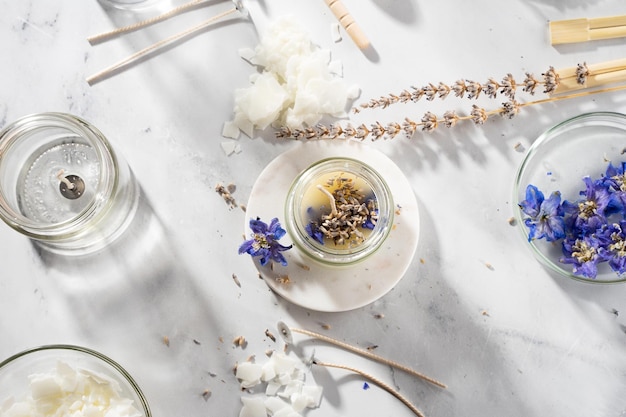This is an overhead color photograph of a white marble countertop adorned with a variety of carefully arranged objects. Centrally positioned is a small clear glass bowl filled with fragrant potpourri, resting on a white saucer. A purple flower, accompanied by several light brown pieces likely from the flower’s center, is delicately placed to the left of the bowl. Above this setup, two sprigs of dried plant stalks add a touch of rustic charm. 

To the left side, there is a round, transparent candle holder or kerosene lamp with a visible white wick protruding from the middle. On the right, a circular glass dish, reminiscent of a petri dish, holds multiple purple flowers of the same type as the one on the saucer. Further to the right top corner, two pairs of wooden chopsticks extend beyond the edge of the table, their wooden surfaces untouched and parallel.

At the bottom left corner of the image, a similarly sized glass dish contains fluffy white objects, possibly some form of dried or decorative material. The various elements spread across the bright, naturally lit marble surface create a harmonious composition, suggesting an aesthetic arrangement potentially focused on sensory appeal, such as scents and textures.